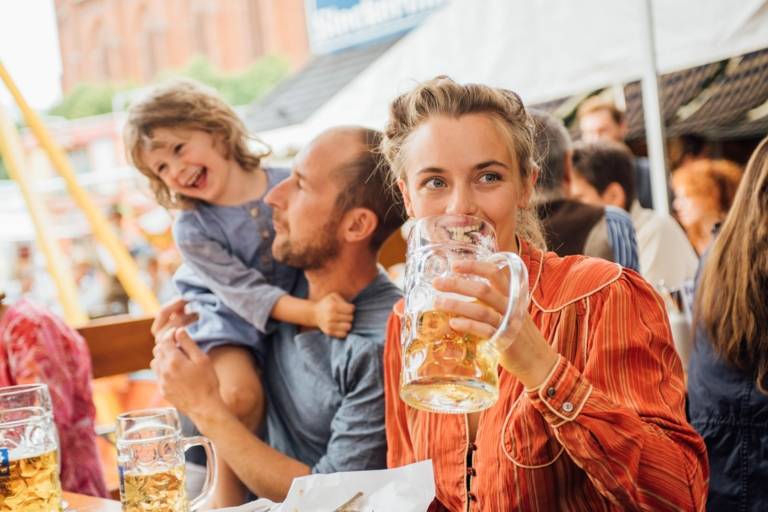This high-quality color photo captures a joyful family scene at an outdoor picnic table. In the foreground, a woman with dirty blonde hair, pulled back, is smiling warmly. She is wearing a red, vertically striped blouse and holding a large, clear glass mug filled with a yellow, tea-colored liquid, possibly beer, close to her mouth. Next to her is a man with balding brown hair, a thin brown beard, and a long nose. He is dressed in a blue shirt and is cradling a small child, who is no more than a couple of years old, in his arms. The child, with dirty blonde hair like the mother, is wearing a blue dress that matches the man's shirt. The child is laughing and gazing off into the distance, while clutching onto the man’s shirt. On the table in front of them, there are additional glass tumblers filled with the same yellow liquid. In the background, other people can be seen enjoying the sunny weather under umbrellas, enhancing the vibrant and cheerful atmosphere of the scene.